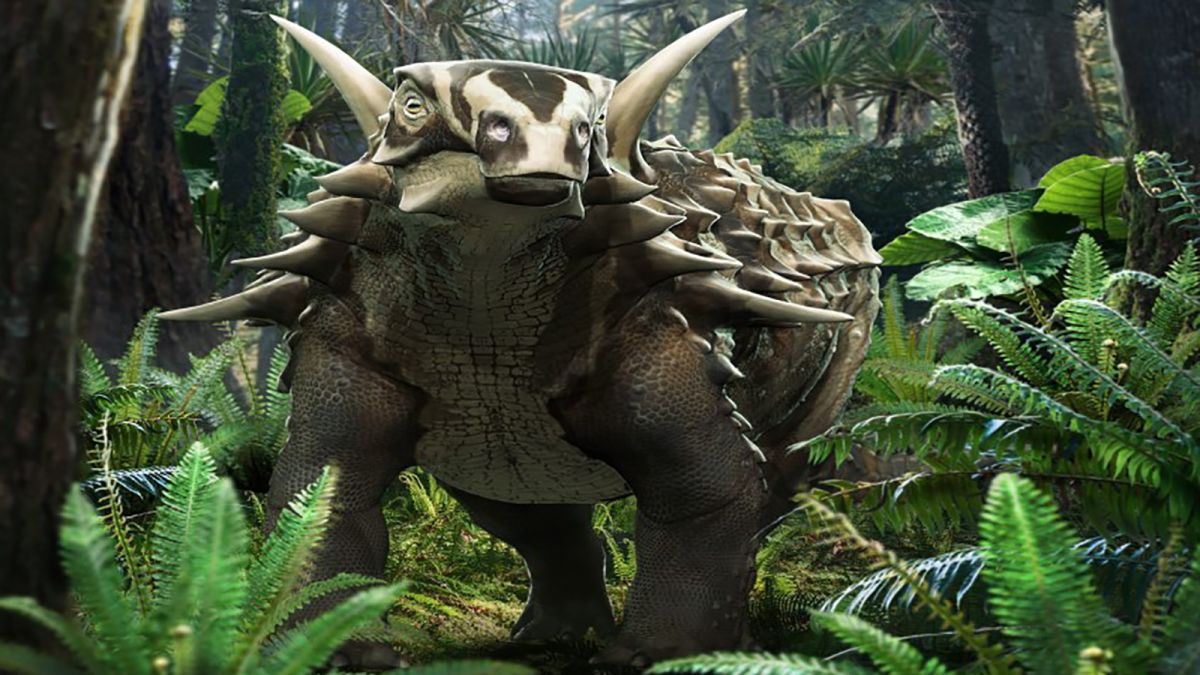In the midst of a lush, tropical forest brimming with vibrant trees and dense, leafy foliage, emerges a fantastical creature that looks as though it stepped out of a sci-fi movie. This formidable beast stands on four powerful legs, with a body that resembles a rhinoceros but adorned with an astonishing array of horns and a peculiar multi-headed appearance. Its skin is a rugged brownish-gray, contrasted by a white chest and belly.

The creature boasts two prominent ivory horns that project majestically from its two distinct heads. Each head has unique features: the forward-facing one bears a cow-like visage with a white face marked by brown patches on the forehead and around the eyes, and a peculiar stitched-looking mouth reminiscent of a snake. The head turned to the side is characterized by half-lidded, snake-like eyes and a wide, grinning mouth. Additionally, an enigmatic third eye peeks from the side, hinting at the possibility of another head altogether.

Smaller horns sprout from the creature's neck, and countless tiny horns cover its robust body, adding to its menacing yet awe-inspiring appearance. This captivating creature stands as a testament to the boundless creativity of the sci-fi genre, harmoniously blending the familiar and the fantastical in a single, striking image.